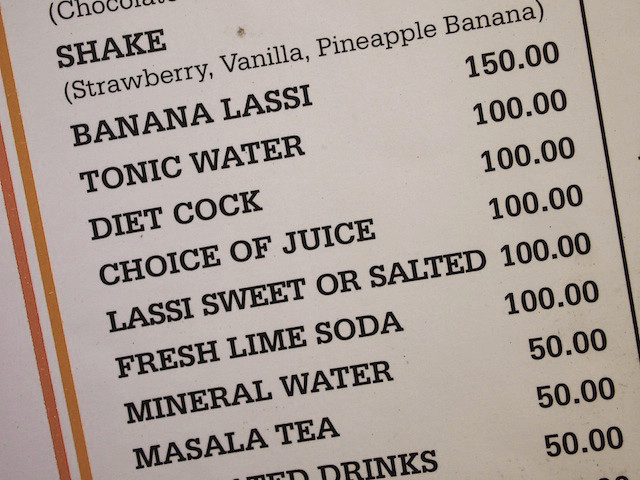The image depicts a photograph of a drinks menu against a white background, featuring text that is angled slightly to the left. The menu is bordered by two vertical yellow-orange lines on the left side and a single black vertical line on the right. The menu items are printed in large black font. At the top of the menu is the word "Shake," followed by a list of flavors: strawberry, vanilla, pineapple, and banana. Below that, it lists "Banana Lassi" priced at 150. The menu continues with "Tonic Water," "Diet Coke," "Choice of Juice," "Lassi (Sweet or Salted)," "Fresh Lime Soda," "Mineral Water," and "Masala Tea." Prices aligned to the right of these items include 100, 100, 100, 100, 100, 150, 50, and 50, respectively, all with two decimal points.